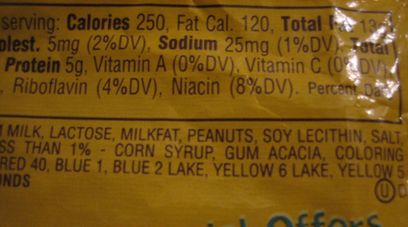This image captures a landscape-oriented Nutrition Facts label set against a mustard yellow background. The text on the label is printed in a clear black font. At the top left corner, the label begins with the word "Serving." Below this, a list of ingredients is provided, which includes: milk, lactose, peanuts, soy, corn syrup, gum acacia, coloring, Blue 1, Blue 2 Lake, Yellow 6 Lake, and Yellow 5.